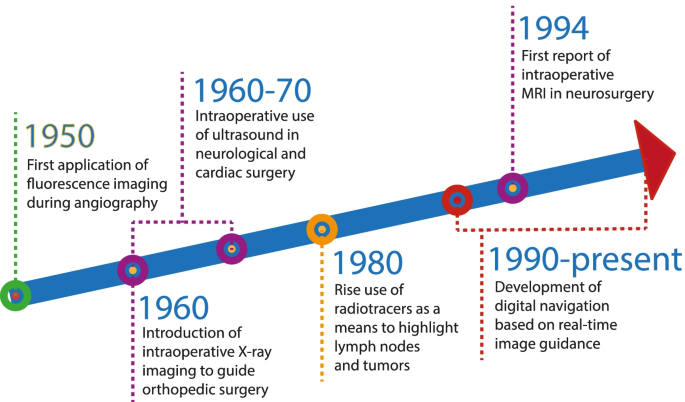This detailed graphic illustration presents a comprehensive timeline of MRI advancements, represented by an ascending blue arrow capped with a red marker. Starting from the left, the first milestone is marked by a green circle at 1950, indicating the "First application of fluorescent imaging during angiography." Moving along the timeline, a purple circle at 1960 notes the "Introduction of intraoperative x-ray imaging to guide orthopedic surgery." Between 1960 and 1970, another purple circle highlights the "Intraoperative use of ultrasound in neurological and cardiac surgery." An orange circle indicates a significant development in 1980: "The rise of radio tracers as a means to highlight lymph nodes and tumors." From 1990 to the present, marked by a red circle, the timeline shows the "Development of digital navigation based on real-time image guidance." Finally, a purple circle at 1994 notes the "First report of intraoperative MRI in neurosurgery," completing the depiction of milestones on this timeline of MRI technology advances.